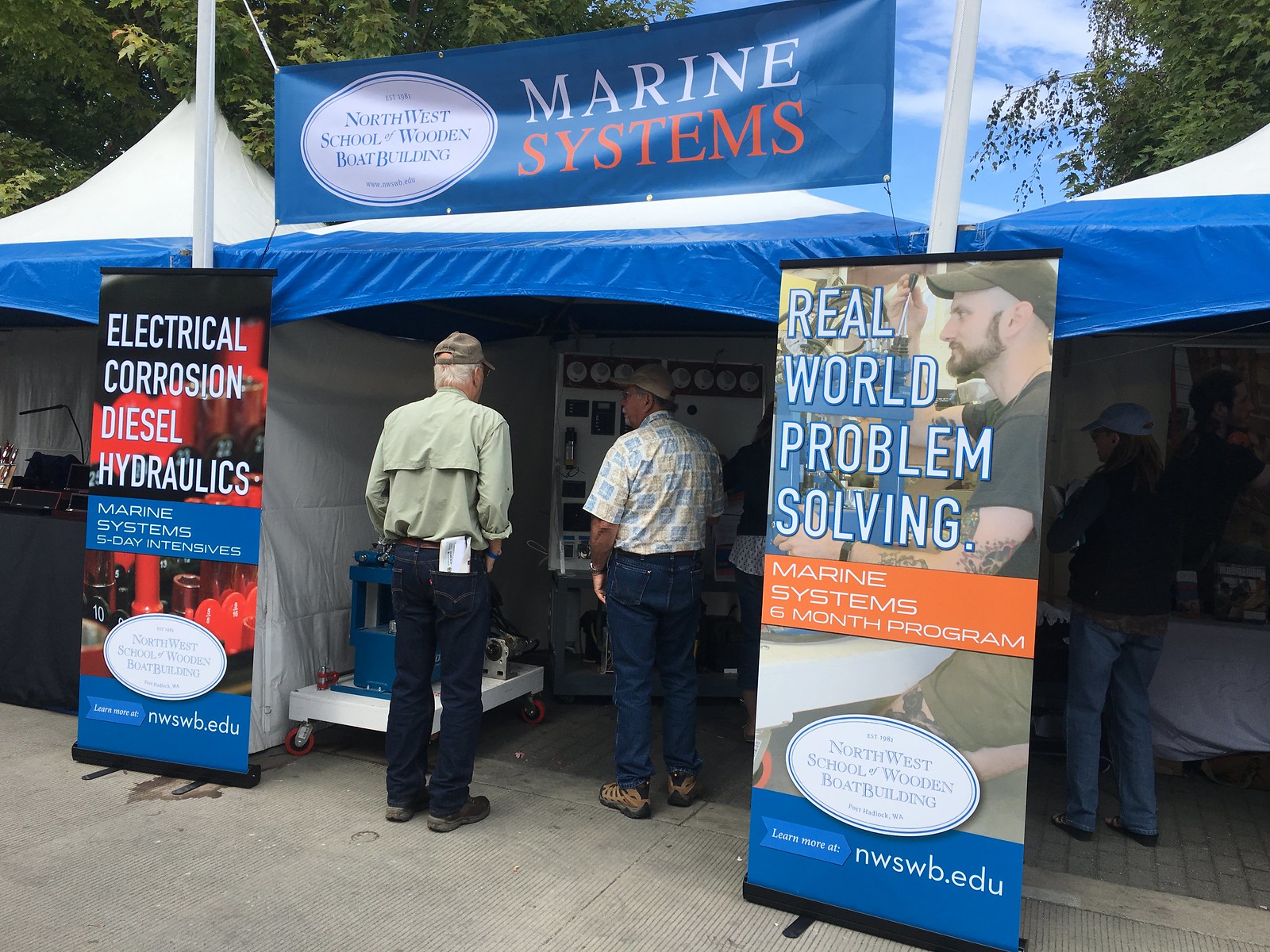The image depicts an outdoor event featuring a large tent set up on an asphalt or concrete surface. The tent, distinguished by its white peaked roof with blue trim along the edges, has three white walls with one wall left open for easy access. Atop the tent, two white poles support a prominent blue rectangular banner, tied at the corners with black and white string. The banner, marked by multiple lines of text, prominently features the words "Northwest School of Wooden Boat Building" and "Marine Systems" in white and orange lettering respectively, alongside a blue oval with additional blue text.

Inside the tent are various displays and tables showcasing products, with people browsing through them. The diverse crowd, dressed in casual attire including closed-toed shoes, shirts, hats, and denim jeans, contributes to the lively atmosphere. In front of the tent, two billboards provide detailed information about the programs offered. The left billboard lists "Electrical Corrosion, Diesel, Hydraulics, Marine Systems Five-Day Intensives," and encourages visitors to "Learn More at nwswb.edu." The right billboard promotes the "Real World Problem Solving, Marine Systems Six-Month Program," and also directs viewers to the same website. This detailed setting highlights the tent as an informational and interactive hub for attendees interested in marine systems and wooden boat building.